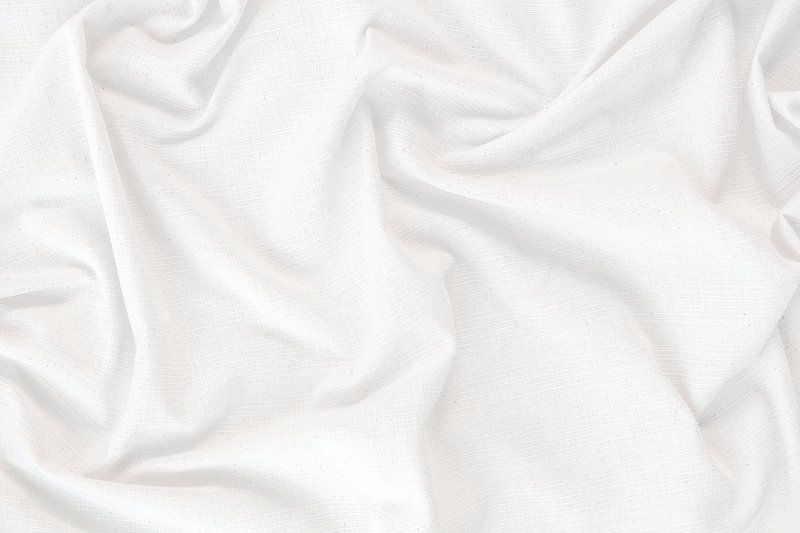This image is a close-up, top-down view of a light-colored, possibly white, silky fabric that is bunched up in various areas. The fabric fills the entire rectangular frame, leaving no background or contrast with other objects. The top right corner has a significant bunching, while the left side shows similar clustering, with the bottom right corner being slightly smoother but still wrinkled. The fabric exhibits gentle folds and shadows, enhancing its texture and imparting a calming effect with shades of white and slight gray tones. The high-quality image captures the tactile softness and irregular folding patterns of the fabric, possibly a blanket or other textile, creating a serene and visually appealing scene.